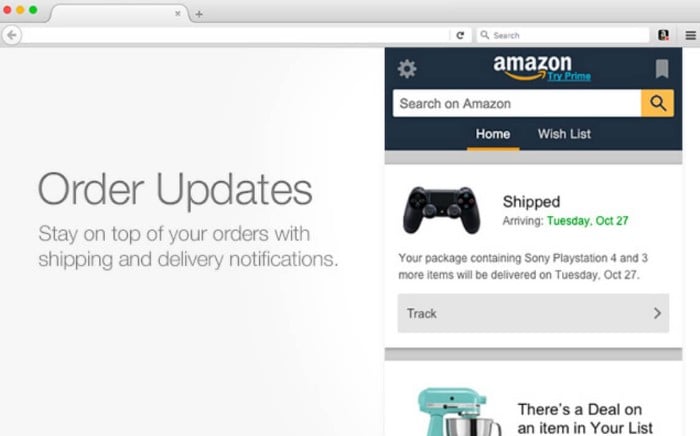This is a detailed screenshot of the Amazon homepage viewed on an Apple Safari browser. The leftmost section features a prominent message in large font that reads "Order Updates." Below this, additional text explains, "Stay on top of your orders with shipping and delivery notifications."

On the right-hand side of the page, the Amazon logo is prominently displayed at the very top within a navy blue box. The logo itself is white, with the characteristic yellow arrow stretching from the "a" to the "z". Adjacent to the logo, there is a clickable blue link that says "Try Prime."

The navy blue header also contains additional icons: a settings icon located at the top left and a bookmark icon found at the top right. The search bar is white, featuring black text for the search query input. The clickable search button is yellow with a black magnifying glass icon.

Below these UI elements, the page content indicates that an item has been shipped and is expected to arrive on Tuesday, October 27th. Accompanying this information is an image of a game controller. The text specifies that a package containing a Sony PlayStation 4 and three more items will be delivered on that date.

Further down, there is an image of an aqua blue stand mixer, alongside a notification that says, "There's a deal on an item in your list." 

Additionally, beneath the search bar at the top of the page, there are navigational buttons for "Home" and "Wish List."